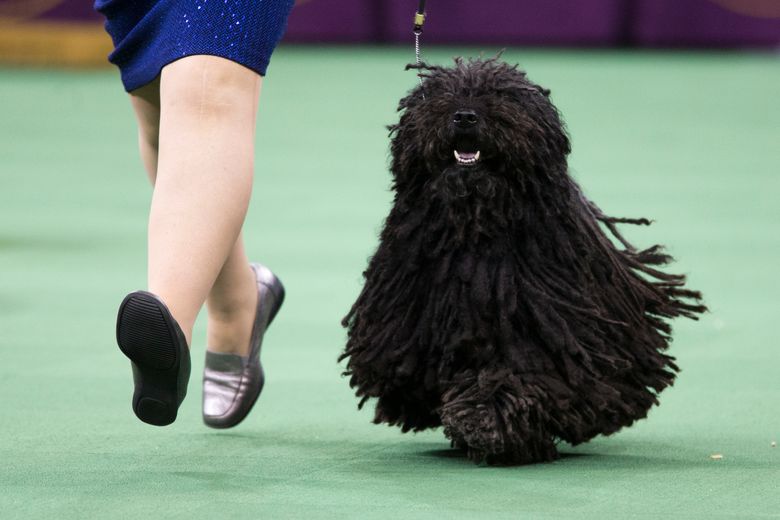In the photograph, we see an elegant woman participating in a dog show, walking a majestic, long-haired dog. The arena floor is a distinct light green, typical of such events. The handler is dressed in a knee-length blue dress and flat silver shoes, adding to her sophisticated appearance. Her attire includes white nylons, enhancing her polished look. The dog, adorned with elaborate, rolled locks of hair that drape to the floor, moves gracefully beside her. Its ornate hair, reminiscent of pompoms, covers its head and eyes, leaving only its black nose, open mouth, pink tongue, and bright white teeth visible. The background is out of focus but suggests the presence of judges at a table, monitoring the event. The photograph captures a detailed and vibrant moment of the dog show.